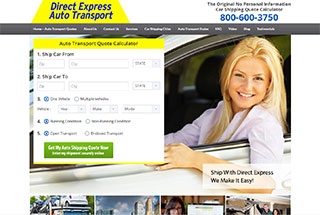Screenshot of an online auto transport service website featuring a white background with various design elements. The main focus is a prominent yellow rectangle with the text "Direct Express Auto Transport" in blue, alongside the phone number "800-600-3750". Below this is a gray bar containing several white icons.

To the right, there's an image of a woman seated in a car, wearing a light pink collared shirt. Adjacent to this image is a white box with a yellow header labeled "Auto Transport Quote Calculator". This section is divided into steps: 

1. First step has several input fields.
2. Second step labeled "Ship Car To", also with several input fields.

Below these steps is a green rectangle with white text.

Further down, a white rectangle with black text reads: "Shop with Direct Express - We Make It Easy". Beneath this are four smaller images: the first shows a car being towed, the second depicts a city skyline, the third is another picture of a woman, and the fourth image is not fully described.